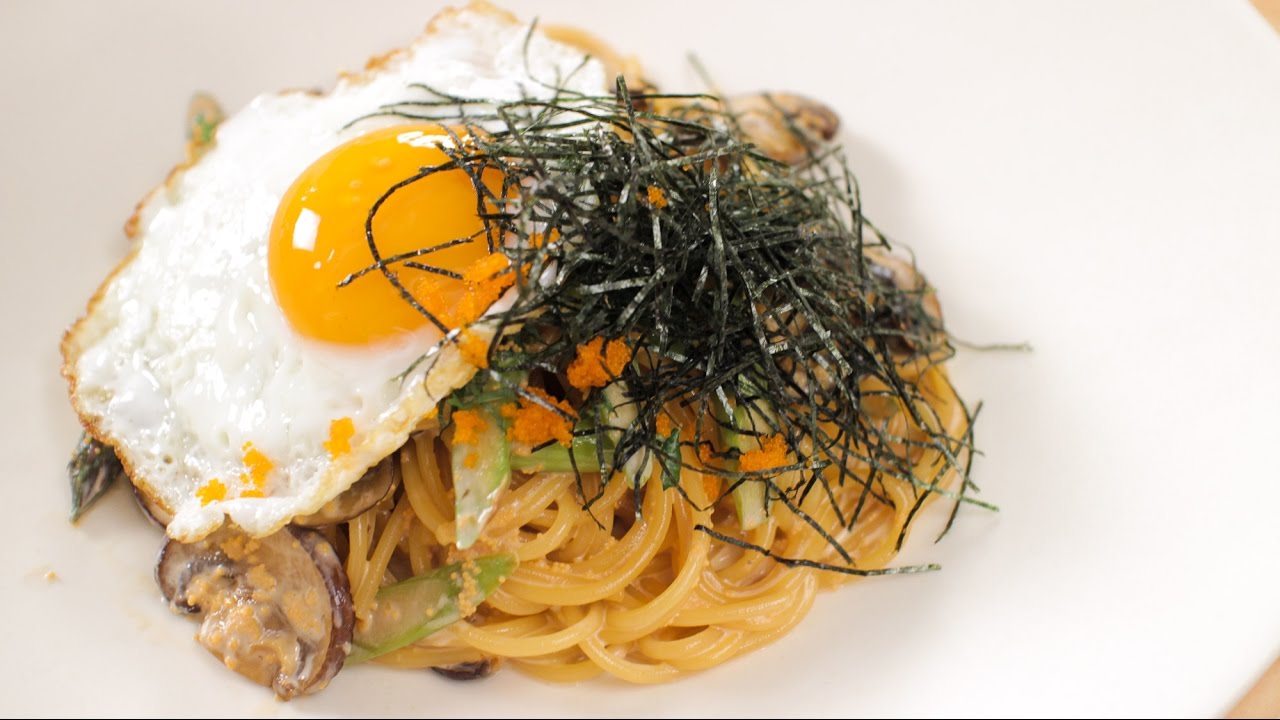This intriguing image features a vibrant and nourishing dish presented on a round, white plate, partly highlighted against a wooden background visible at the edges of the composition. At the heart of the dish lies a golden, sunny-side-up egg with a soft, runny yolk, slightly crusted on the outer edges. Beneath the egg is a bed of yellow, spaghetti-like noodles, possibly made from squash, giving the dish a unique, creamy appearance without a distinct sauce. To the side of the noodles, you can find a medley of vegetables including bright orange carrots, a sliver of mushroom with a reddish tint, and a few stalks of asparagus. A touch of dull green seaweed or sprouts adds a final garnish, intertwining with potential bits of celery and caviar. This amalgamation of ingredients not only makes for a visually compelling dish but also suggests a nutritious and diverse culinary creation.